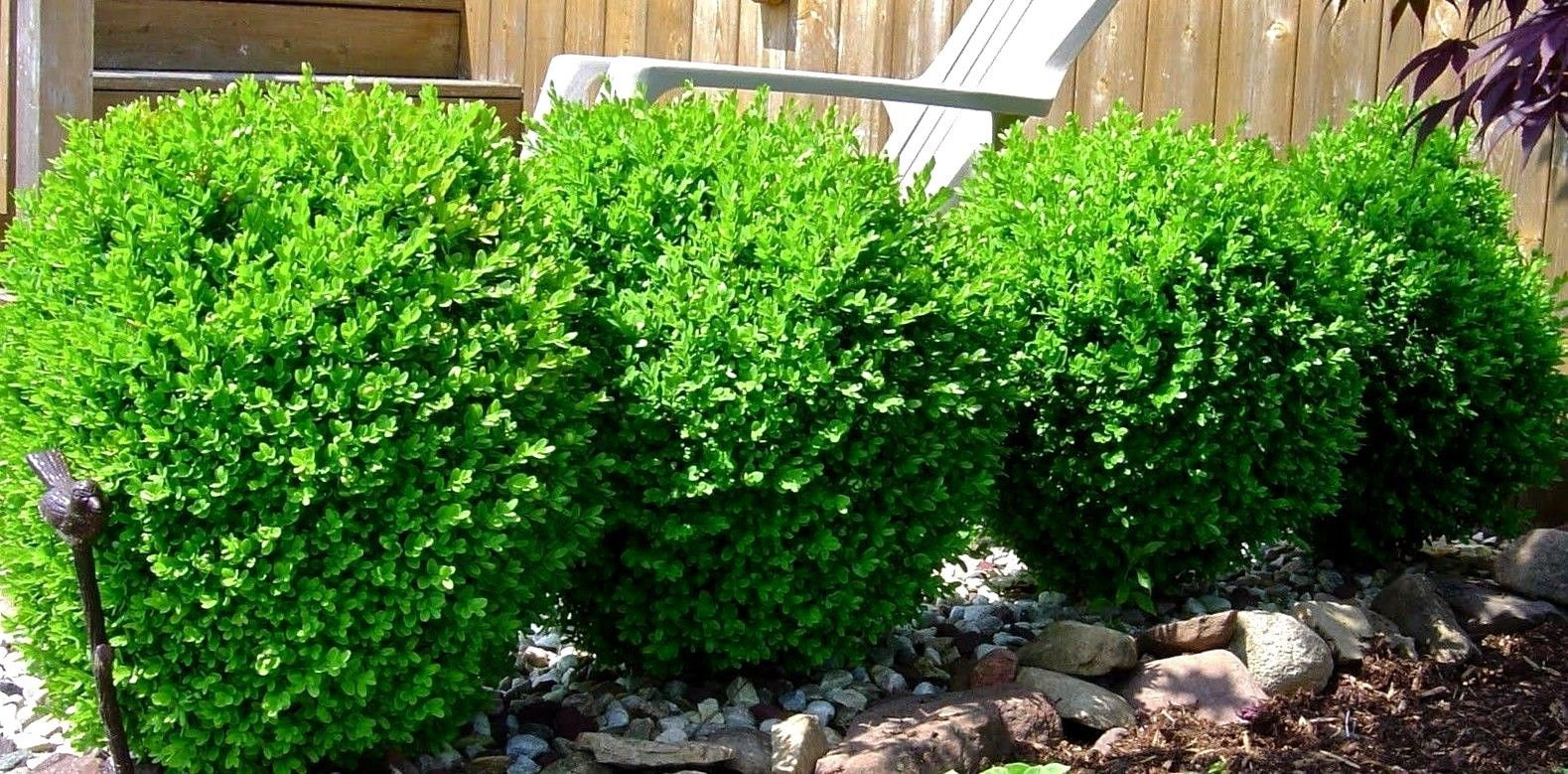This is a detailed color photograph of a landscaped area, likely part of a residential or office building's yard. The main focal point is a row of four green, round, boxwood shrubs, each growing freely without being trimmed into a specific shape. These shrubs are a couple of feet tall, and they sit on a bed of rocks, serving as a distinct border for the garden area. Behind the shrubs, there is a white plastic Adirondack lawn chair bathed in sunlight, with the foliage partially obscuring the chair's legs, showing only its armrests clearly. A wooden fence forms the backdrop, and in the upper left corner of the image, there's a partial view of a wooden staircase with two visible steps, adding an element of depth to the scene. Additionally, in the front, there is a mix of mulch and a series of large stones that outline the garden bed. A post topped with a bird figure and a black object protruding from the ground are also visible, contributing to the garden's decorative elements. Overall, the image captures a serene and well-maintained outdoor space.